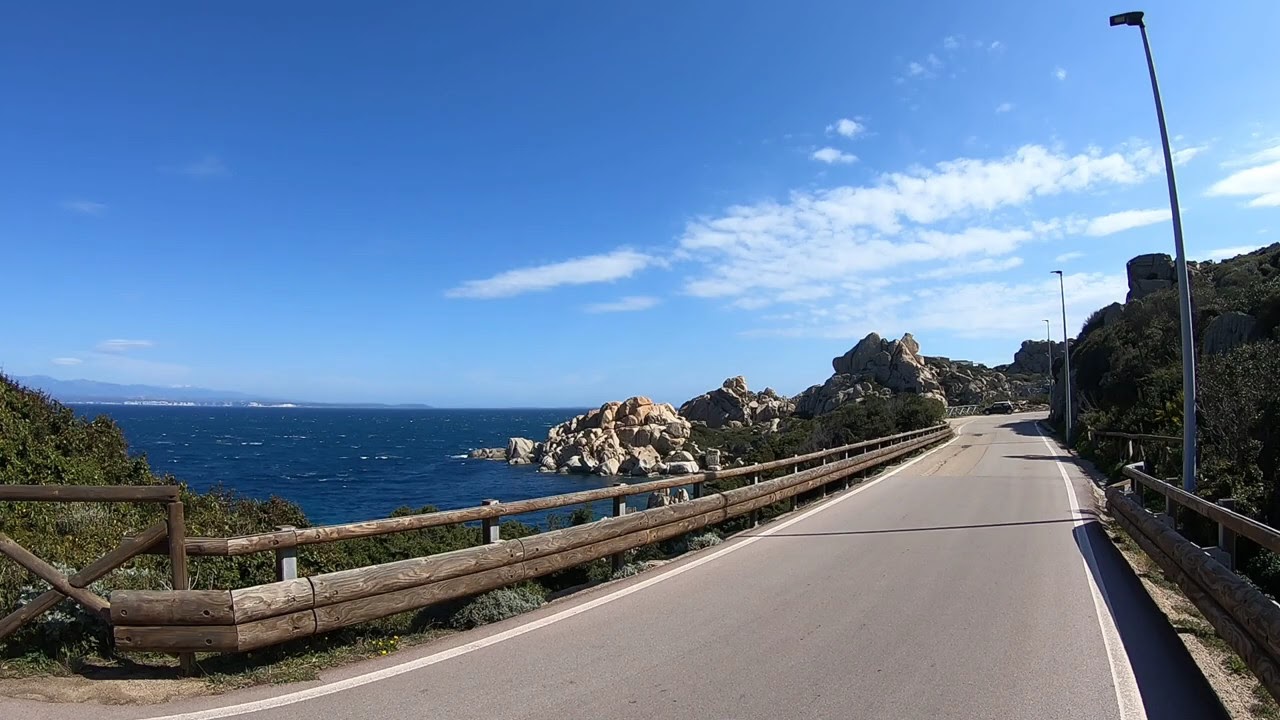This photograph captures a serene coastal scene on a sunny day with a bright blue sky adorned by a few wispy clouds. The road in the foreground is narrow, likely a single lane, and appears to be made of asphalt, bordered on the left by wooden guardrails that hint at a quaint, rustic charm. On the left side of the road stretches a vibrant blue ocean meeting a rocky, unsandy shoreline; jagged rocks protrude out into the sea, and a rocky cliff rises nearby. The far left reveals the faint outline of distant land or a mountain line shrouded in hazy fog, suggesting it could be a bay area. There are streetlights positioned on the right side of the road. Vegetation covers the hill on the road's right side, adding a touch of greenery to the landscape. Further down the road, there is a car parked at a pull-off area on the left, and the road continues straight before curving off to the right in the distance.